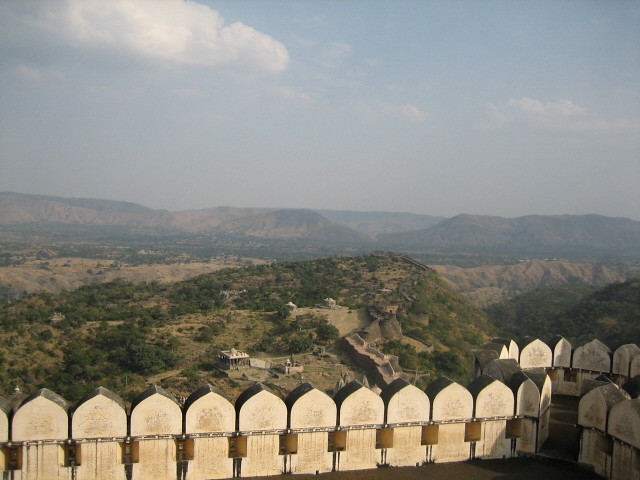This is a detailed outdoor photographic image captured during the daytime from the vantage point of someone standing on a terrace or castle-like structure. The terrace is lined with about 12 to 13 pointed white arches that resemble the top of a tower, giving the appearance of a continuous fence or barricade. Below, the foreground of the image features this extensive stretch of white, off-white arches. 

In the mid-ground, a lush, green valley unfolds, adorned with rolling hills and clusters of buildings. Some buildings are distinct with architectural elements like turrets and cupolas, predominantly white in color and nestled among the greenery.

The background extends into a sweeping panorama of brown and tan mountain ranges, adding depth to the composition. The mountains run horizontally from left to right and have an aspect reminiscent of the Great Wall of China due to a visible wall-like structure. The sky above is a gradient of blue, fading to a lighter white due to cloudiness, suggesting an overcast day yet still bright with sunlight. The overall setting creates a magnificent view of natural and man-made beauty, captured thoughtfully in this image.